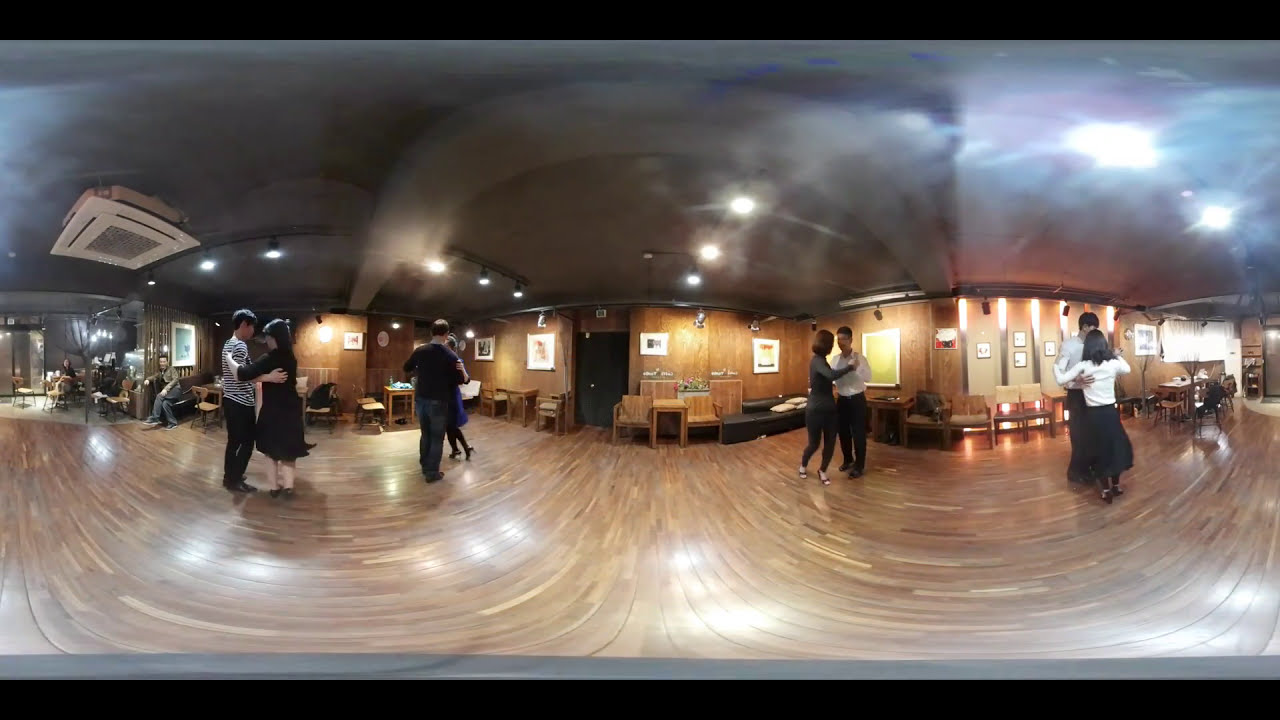This color indoor photograph, captured with an extreme fisheye lens, offers a panoramic view of a dance hall. The distorted and flattened perspective reveals four couples dancing on a brown hardwood floor. The ceiling is adorned with a network of black metal bars or tracks housing bright white light fixtures. 

In the middle of the image, a seating area with long upholstered benches surrounds a doorway leading to another room. The walls, also wooden and brown, are decorated with framed images. To the right, more seating areas, tables, and an array of framed pictures are visible. 

On the left side, an HVAC ventilation unit is ceiling-mounted. People sit in the background, particularly to the left and center of the image. The dancers appear to be in ballroom type embrace, likely enjoying themselves or perhaps participating in a professional ballroom event. Out of the four couples, notable are the man in a black and white shirt and black pants dancing with a woman in a black dress, and another pair where the woman wears a purple dress dancing with a man in a black shirt and blue jeans.